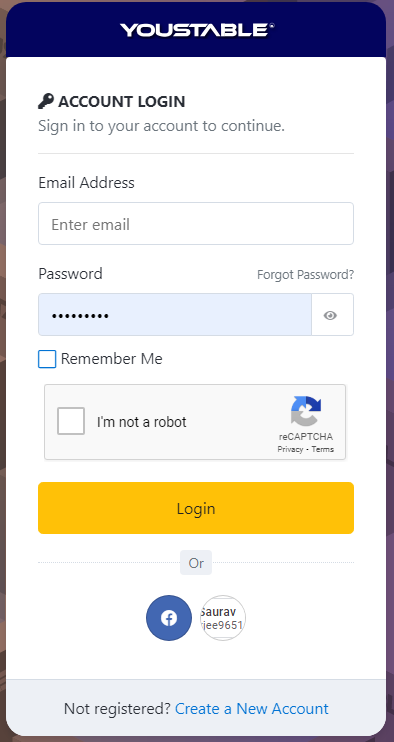The screenshot displays the login screen of the uStable app. At the top, there's a dark blue-purple header that contains the uStable logo. Below this header, the background is white. In the upper section, there is a black key symbol next to the text "Account Login." Below this, in a slightly darker gray color, is the instruction: "Sign in to your account to continue."

The login form includes an email address field and a password field, both clearly labeled. Above the password field, there is a "Forgot Password?" link. Below the password field, there's a "Remember Me" checkbox. 

Towards the bottom of the login section, there's a CAPTCHA checkbox labeled "I am not a robot." The login button is prominently displayed in a yellow color with black text. 

Underneath the login button, the options "Log in through Facebook or Twitter" are presented. Lastly, in dark gray text, there is a prompt that reads "Not Registered?" with a clickable "Create New Account" link in blue to allow for account creation.